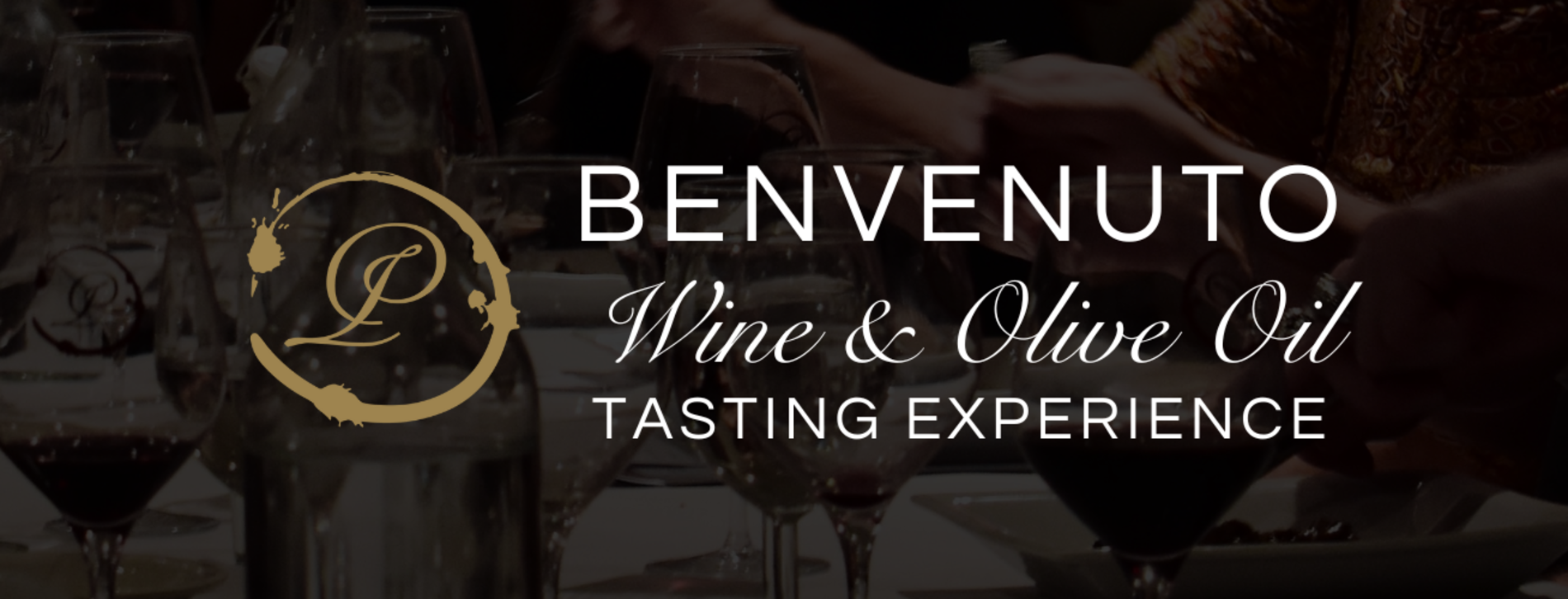The image is a horizontal rectangular banner promoting a wine and olive oil tasting experience. The background is a transparent black overlay with a faint, blurred photograph of a table setting featuring wine glasses, bottles, and white tablecloths. On the left center of the banner, there's a gold circular logo resembling a wine ring stain, with a script emblem inside. To the right, bold white sans-serif text at the top reads "BENVENUTO" in all capital letters. Below it, in white script text, the words "wine and olive oil" are displayed, followed by "tasting experience" in slightly smaller bold sans-serif text. A woman's hands handling some items on the table are faintly visible in the right-hand side of the background.